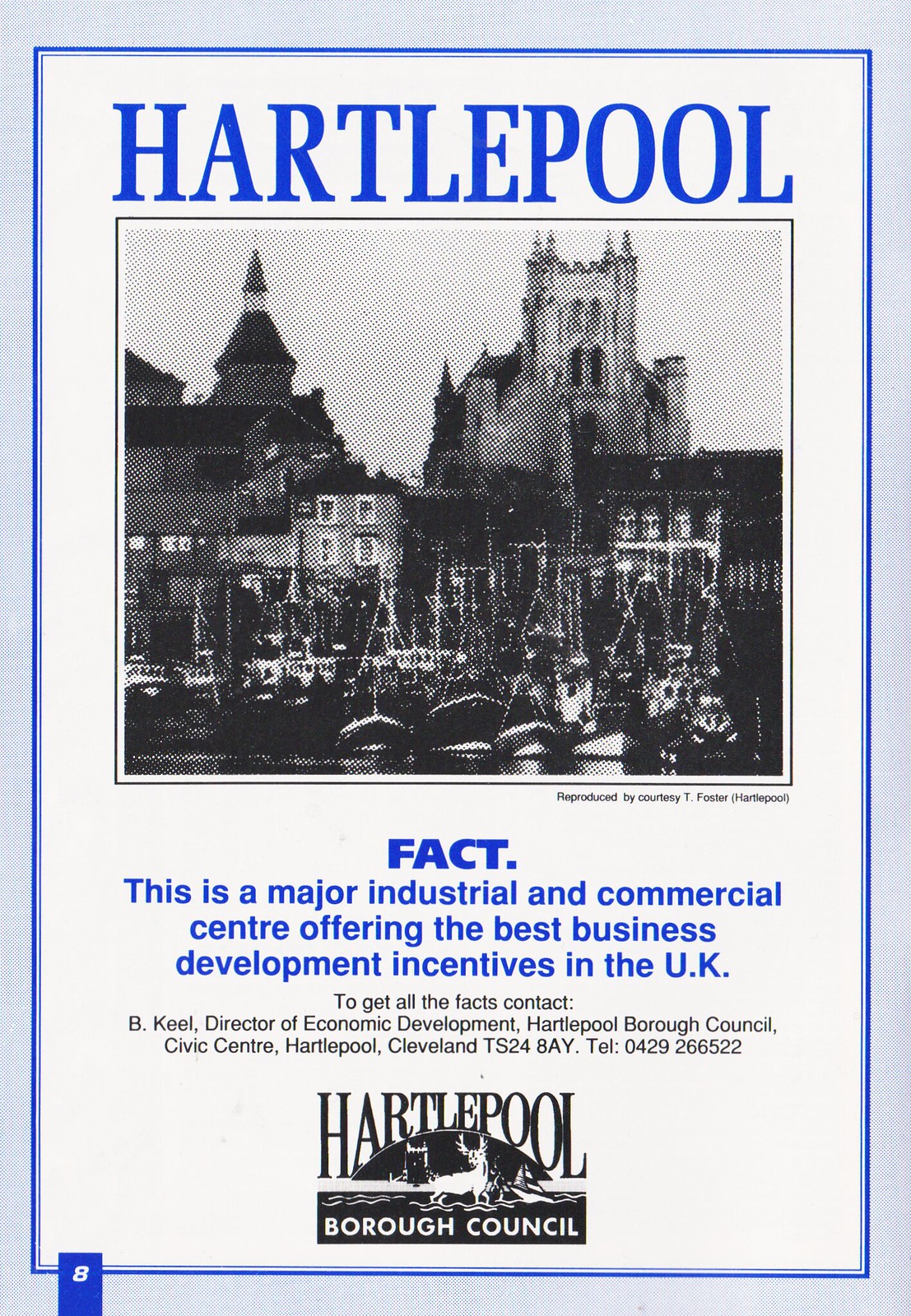The vertically oriented advertisement features a central title in blue text reading "Hartlepool." Below the title is a black-and-white image that has a textured, pixelated appearance, reminiscent of a newspaper print. The image depicts a dock area in Hartlepool, with numerous boats closely clustered together along the waterfront. In the background, a variety of buildings are visible, including what appears to be a cathedral or a castle. The image is credited beneath it with the note, "Reproduced by Courtesy T. Foster Hartlepool." Under the photograph, a block of blue text states: "FACT: This is a major industrial and commercial center offering the best business development incentives in the UK." Below this, it continues with contact information: "To get all the facts, contact B. Keele, Director of Economic Development, Hartlepool Borough Council, Civic Center, Hartlepool, Cleveland, TS24." A phone number is also provided. The entire advertisement is bordered by a light blue frame, and a small number "8" is located in the lower left corner, indicating the page number.